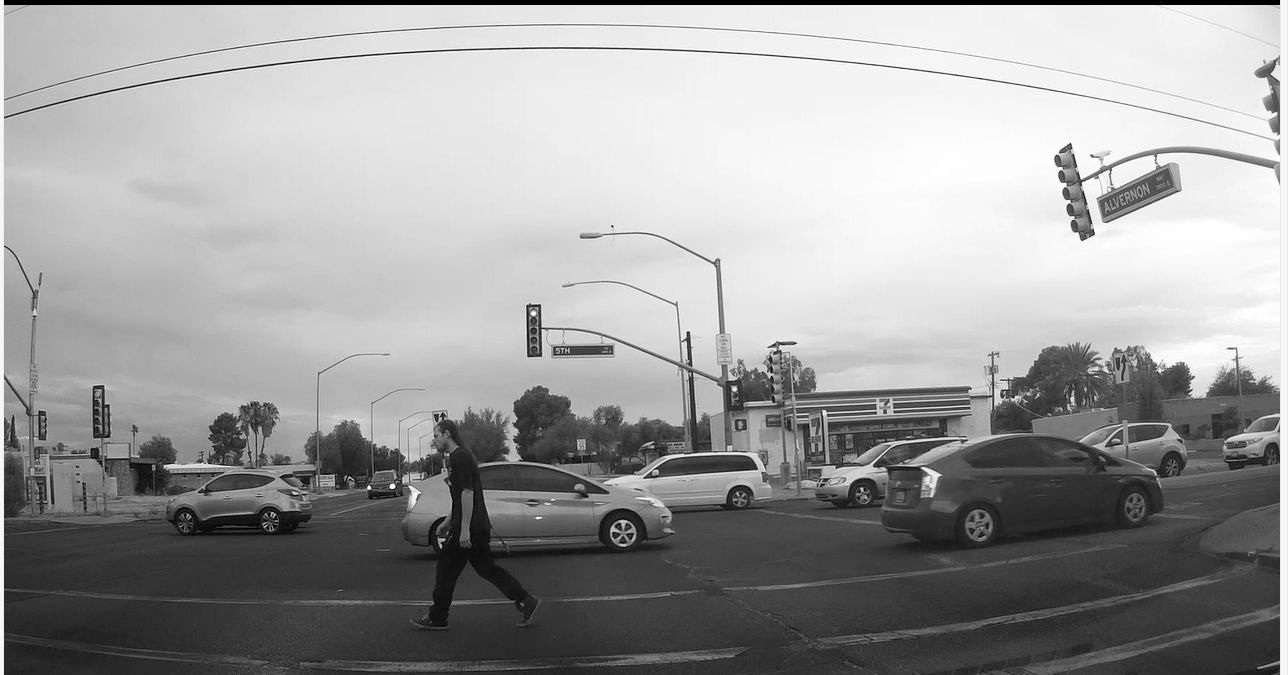This black and white, wide-angle photo captures a bustling intersection from the perspective of a car's windshield. Central to the scene is a man dressed in black, with long hair, walking across the street towards the left side of the frame. The intersection is busy with cars moving in both directions—the most prominent one directly in front of the viewer's car, and another passing under a stoplight to the right. Elevated above the intersection, a stoplight with attached cameras and a street sign faces the left side of the frame. The curvature of electrical lines is noticeable due to the photo's wide-angle distortion. A 7-Eleven sits prominently to the right in the background, its lights illuminating the parking area. Additional light poles, trees, and buildings line the street, emphasizing the typical urban setting of what appears to be a U.S. city, evidenced by the make and model of the cars.